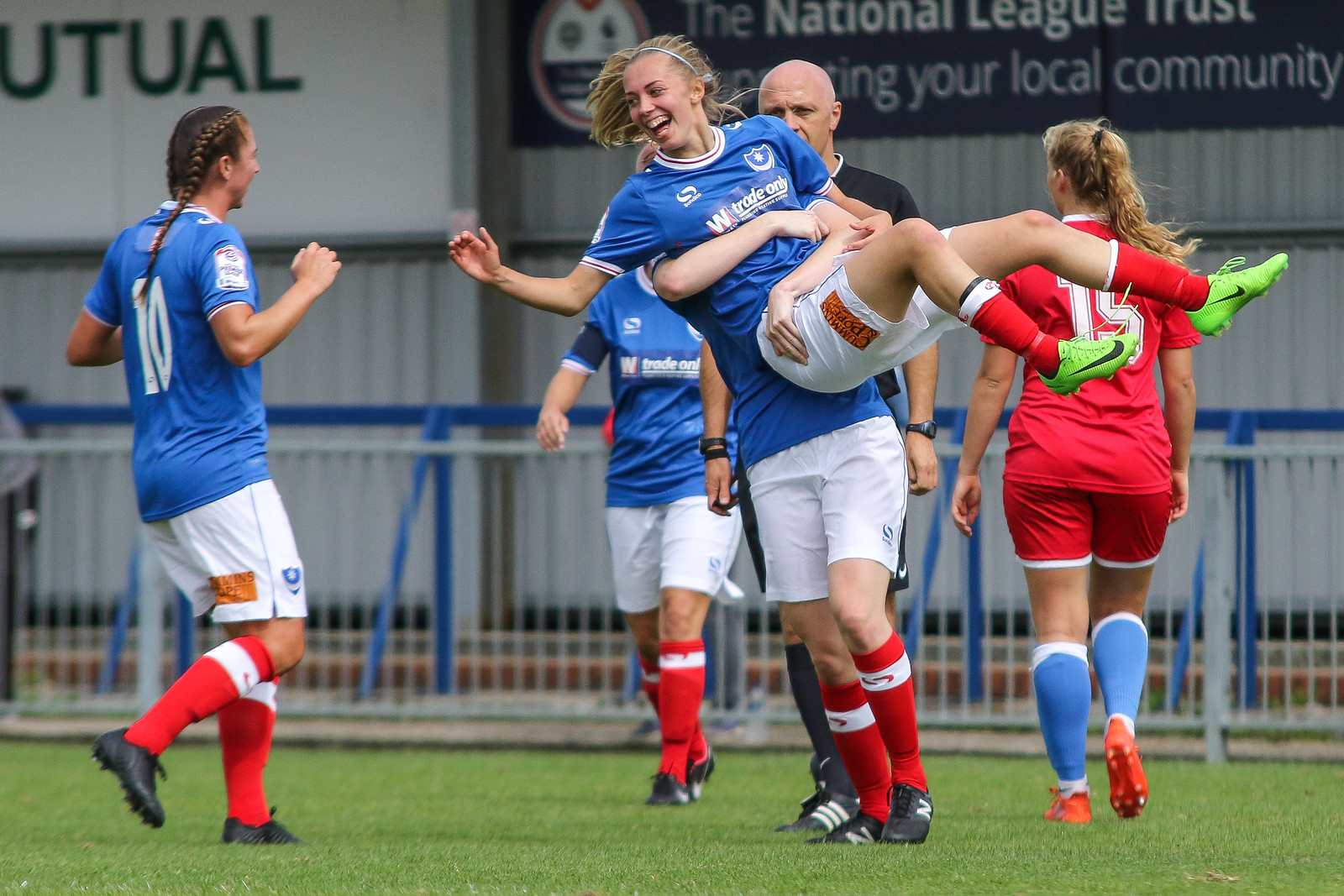In this vibrant photograph capturing a moment from a women's soccer match, four players in blue shirts and white shorts are at the center of attention, celebrating an important event in the game. One of the blue-clad players, hoisted joyfully in the air by a teammate, beams with a broad smile while reaching out for a high-five from another teammate rushing toward her. Nearby, a player in a red shirt, red shorts, blue socks, and orange cleats marked with the number 15 walks away from the celebratory group, her long blonde ponytail swaying with her stride. In the background, a referee in a black shirt is partially visible, observing the scene over his shoulder. The action unfolds on a green turf field bordered by a low, gray fence reminiscent of a bike rack, with partially visible advertisements adorning a backdrop structure, hinting at local community support.